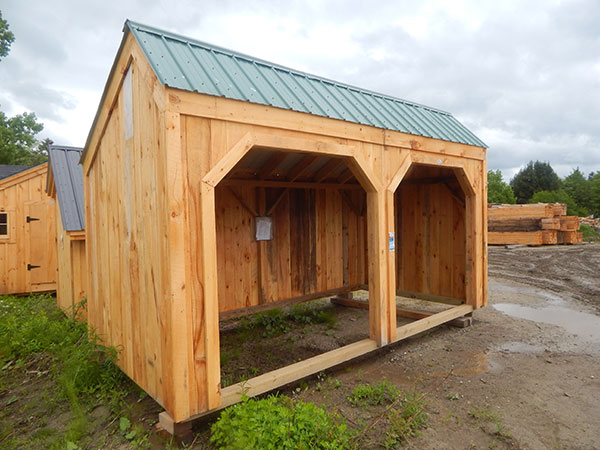The image depicts an active construction site characterized by a muddy, spotty terrain interspersed with patches of grass or weeds. Central to the picture is a small wooden edifice, reminiscent of a shed, featuring two unfinished door frames shaped like half octagons. The edifice is constructed from raw, light-colored wood, possibly pine, with a green sloped metal roof. Nearby, two similar structures are visible, indicating multiple builds in progress. The site resembles a lumber yard, with stacks of timber positioned against trees in the upper right background. The ground is muddy with visible puddles, suggesting recent rainfall. The sky is overcast, and in addition to the construction, there are scattered wood materials in the distance. The area seems designed for constructing prefab small buildings, potentially for parking small vehicles like tractors or golf carts.